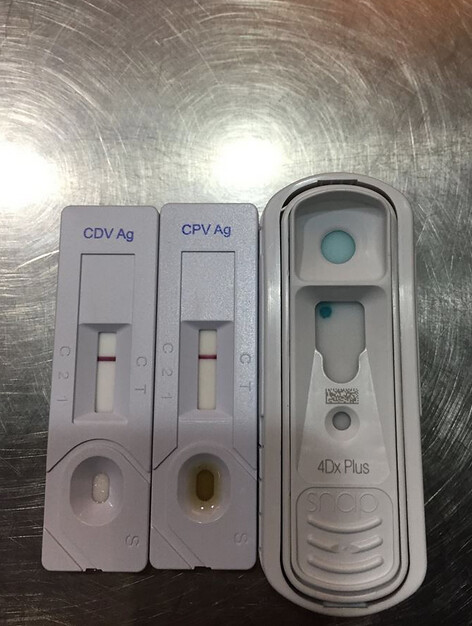This photograph depicts three plastic testing devices, presumably used in a chemistry setting, arranged on a metallic table. The table reflects two lights above, casting a distinct shine onto the plastic devices below. Positioned in the bottom 65% of the image, the two devices on the right are nearly identical. These light blue-gray rectangular items feature "CDVAG" in blue ink on their top surfaces. Below this text, a small, indented box gives way to a white strip marked with "O, 2, and 1" on the right and "O and T" on the left, both pointers currently set to "O". Further down, each device has a curved section containing an egg-shaped indentation filled with a white substance, and the one on the right contains an orange substance that resembles iodine.

Contrastingly, the device on the left is fully gray and of a different design. It is larger and features rounded edges. Its top and bottom sections are conspicuously curved, resembling a phone. The bottom part of this device includes a thumb rest marked with "4DX+", above which is a small circle with an intricate rectangular design. A circular groove leading into a black area with a blue dot on the right corner is also present, followed by what looks like the head of a phone with another blue dot. This meticulous arrangement and distinct features easily differentiate the gray device from its nearly identical light blue-gray counterparts on the right.